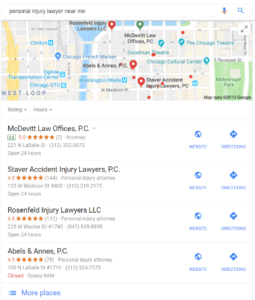This image depicts a search result page from a maps application. At the top, there is a small text bar with the search query "personal injury lawyer near me." Below the search bar, a map is visible, displaying streets, highways, and a body of water, potentially a river or lake. 

Several red pins on the map indicate the locations of the search results listed beneath it. The first result is for "McDevitt Law Office's PC," which appears to have a five-star rating. Next to this result, there are links labeled "Website" and "Directions." Additionally, there is a small green rectangle indicating that this is a paid advertisement. 

The second result is for "Staver Accident Injury Lawyers PC," which has a rating of four-point-something stars. This entry also includes links for "Website" and "Directions." Following this, "Rosenfeld Injury Lawyers LLC" is displayed with a similar rating of four-point-something stars and the same accompanying links. 

Finally, "Abel's and Anne's PC" is listed with a 4.5-star rating, along with the "Website" and "Directions" links. At the bottom of the search results, there is an option in blue text to view "More places."